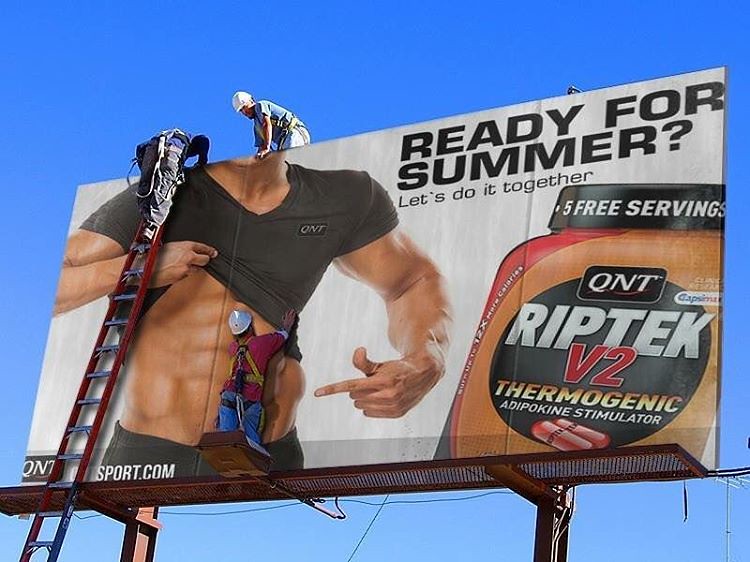In this photograph, several men are actively working on applying a large, promotional billboard. The billboard showcases an image of a muscular man, depicted from his chin to his waist. He is wearing a black shirt, lifted to reveal his toned stomach, which he points to with his left hand while his right hand holds up the shirt. Prominently featured next to the man is a container labeled "Riptek B2 Thermogenic," highlighting an offer of "five free servings" displayed on its cap. The billboard's bold, black text reads, "Ready for summer? Let's do it together." In the bottom left corner, the website "sport.com" is listed.

A man stands on a ladder, leaning over the top edge of the billboard, although the base of the ladder is out of view. Another worker is visible from the hips up, positioned behind the billboard and leaning forward, aligning his torso near the chin of the man portrayed. A third individual focuses on smoothing out the lower portion of the billboard, ensuring the material lies flat against the man’s stomach in the advertisement. The scene captures the teamwork and effort involved in setting up this eye-catching summer fitness promotion.